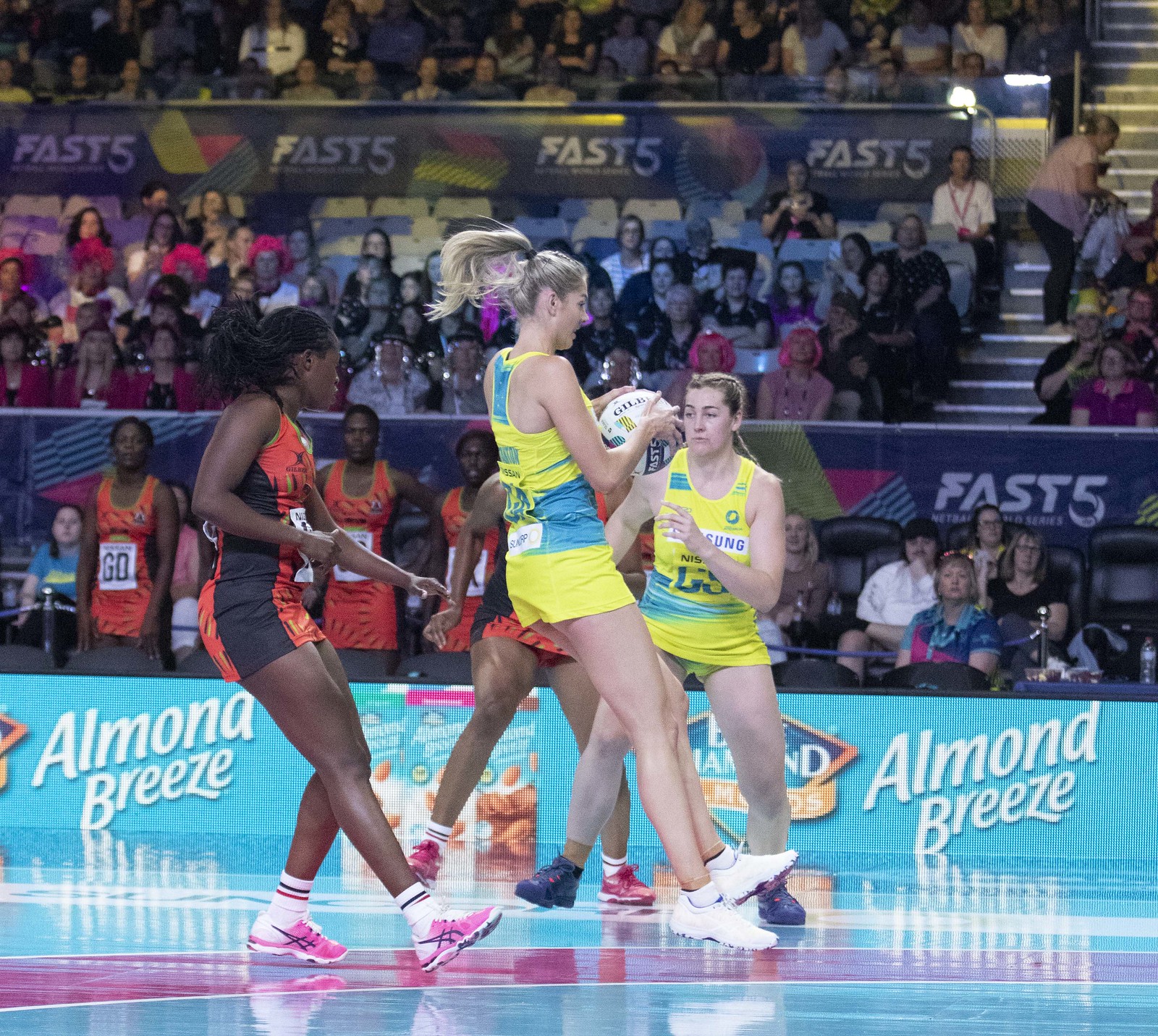In the indoor arena of a flashy blue and pink court, a volleyball match unfolds with intensity. The two competing teams stand out vividly; one team clad in blue and yellow uniforms, the other in red and black. Central to the action is a tall, blonde woman in the blue and yellow attire, captured in mid-jump, clutching a white volleyball. Her blonde hair, tied back in a ponytail, flows behind her as she descends. Beside her, another teammate in the same vibrant uniform, her braided blonde hair visible, readies herself for the next play.

Approaching these two athletes are two African-American women from the opposing team, dressed in sleek red and black jerseys, their pink sneakers adding a pop of color to the scene. Behind the players, a large banner with "Almond Breeze" can be seen, partially obscured by teammates and spectators. The stands are filled with an engaged audience, including another player in a red and black outfit, marked with the number 60.

The gymnasium’s glossy wooden floor is painted in striking shades of aqua blue with pink stripes, enhancing the vibrant atmosphere. The "FAS5" banner hangs prominently, reinforcing the event’s bustling energy. This image captures the dynamic and colorful essence of a high-stakes volleyball game, brimming with athletic prowess and spectator enthusiasm.